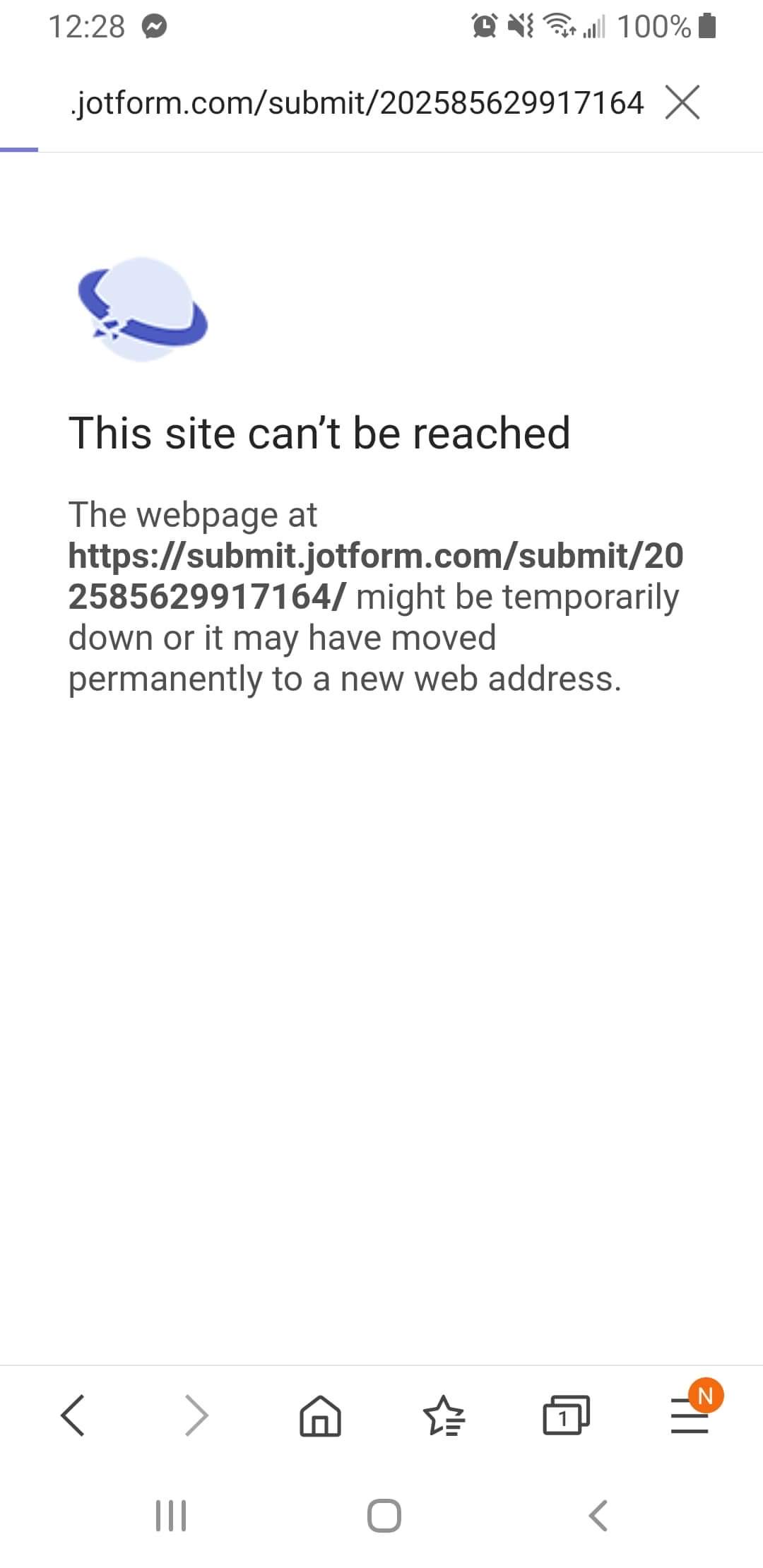The image displays a webpage error message against a white background. At the top, the text "1228" appears in black, accompanied by a small gray chat icon featuring a white lightning bolt in its center. To the right, several icons are lined up: a clock, a muted volume symbol, signal bars, volume bars, "100%" followed by a fully filled black battery icon.

Below this, in black text, is a URL: "jotform.com/submit/202-585-629917164" next to a large gray "X". A thin horizontal line extends from left to right, starting with a small blue section.

Underneath, in black font, it states, "This site can't be reached." This message is followed by additional text explaining that the webpage at "https://submit.jotform.com/submit/202-585-629917164" might be temporarily down or may have moved to a new web address.

In the center of the image is a light blue circle resembling the planet Saturn with a darker blue ring around it, floating against the white background.

At the bottom of the image are navigation icons: a black left arrow, a gray right arrow, an outlined house icon, an outlined star with three horizontal lines, two outlined gray boxes with a number "1" inside one, the menu bars represented by three horizontal lines, and an orange circle with a white "N" above the menu icon.